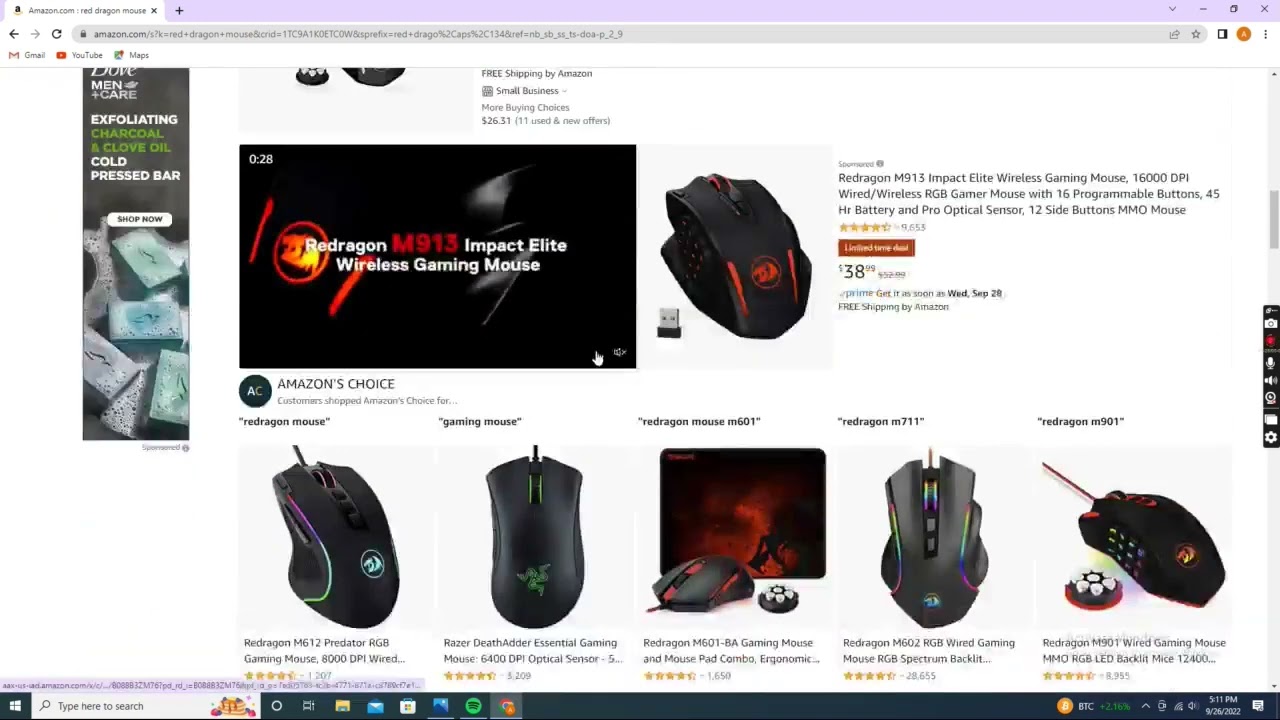A screenshot of a webpage, likely from amazon.com, is displayed. The page features a distinctive purple bar at the top, with navigation options for Gmail, YouTube, and blogs along its sides. On the left section, there is a featured product: "Dove Men+Care Exfoliating Body Bar with Charcoal and Clove Oil," which is available for purchase immediately. 

On the right, a partially scrolled section showcases the "Redragon M913 Impact Elite Wireless Gaming Mouse," priced at $38. The mouse is highlighted as Amazon's Choice and has an approximate 4.5-star rating. Below this product, there are five additional gaming mice options listed, most appearing to have cords, though a few may be wireless. This detailed display invites gamers to browse and purchase their preferred gaming accessories directly from the site.